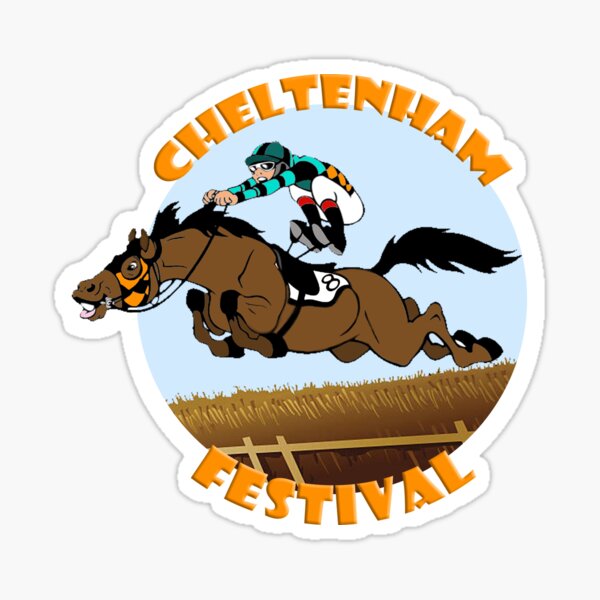The image is a digital, cartoon-like logo for the Cheltenham Festival, set against a gray-white background. The logo is mostly circular but has some detailed protrusions on the top, bottom, and left sides. The words "Cheltenham" and "Festival" are prominently displayed in large, puffy, orange letters arcing over the top and bottom of the image. At the center, it depicts a jockey in mid-air, seemingly having just bounced off the saddle of a leaping brown horse with the number eight on its left side. The horse, which has a black tail and hooves, an orange face halter, and an open mouth with wide eyes, looks excited as it jumps over a fence into a field of brown grass. The jockey is dressed in white jodhpur pants, black boots, a turquoise and black striped shirt, a teal helmet, and white goggles, adding vibrant color to the scene. Dark brown hay can be seen underneath the horse and along the fence.